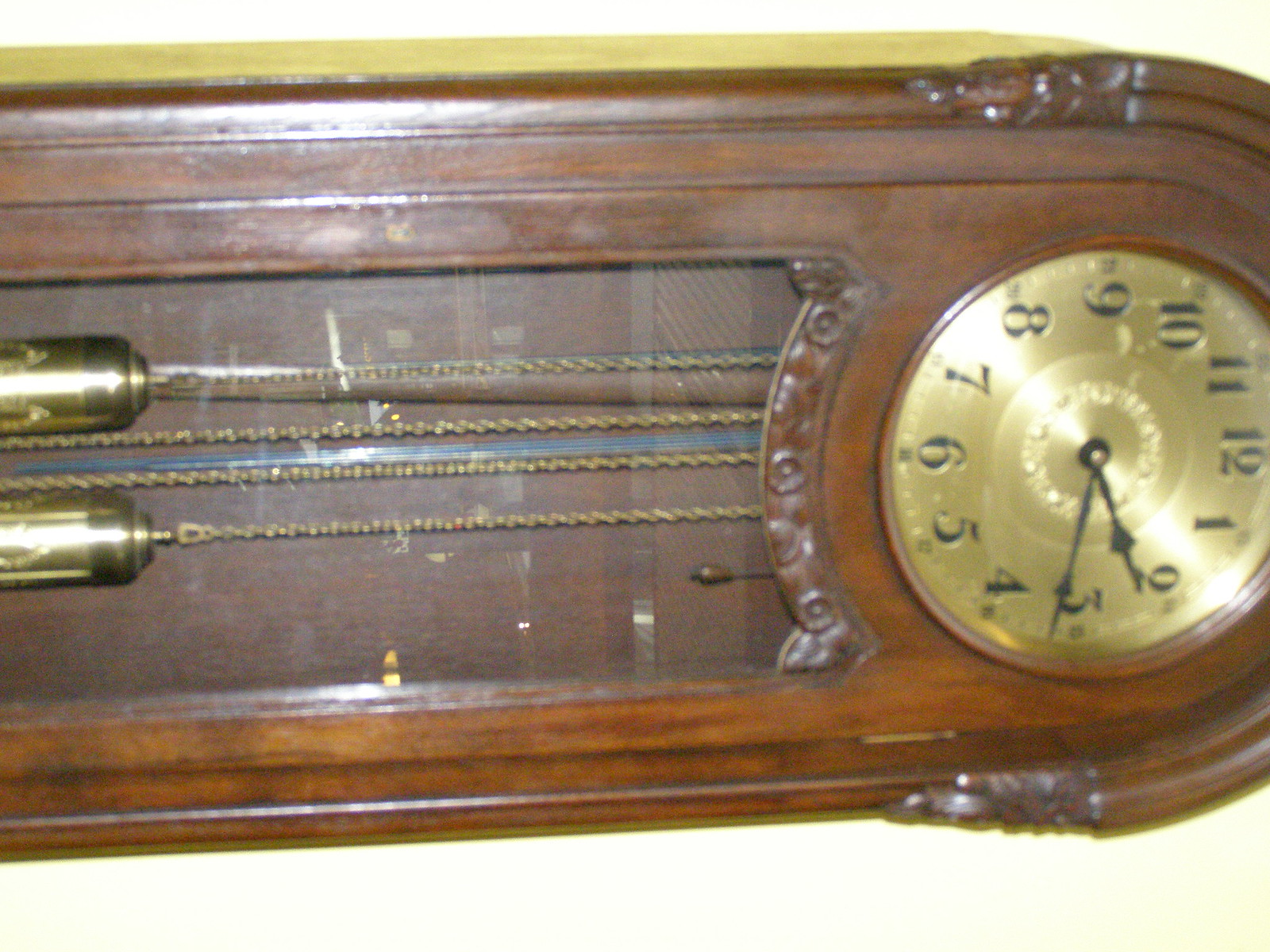This photograph features a rotated image of a classic grandfather clock in a landscape orientation, meaning the width exceeds the height. Constructed from a dark oak or maple-hued wood, the clock showcases intricate detailing, particularly at the top arc. Below the round, gold clock face, a glass pane reveals the clock's internal mechanism with weights suspended on gold or brass chains. The clock face is adorned with traditional black numerals, and the black clock hands indicate the time as 2:17. Overall, the detailed craftsmanship and rich wooden tones highlight the elegance and timeless nature of this grandfather clock.